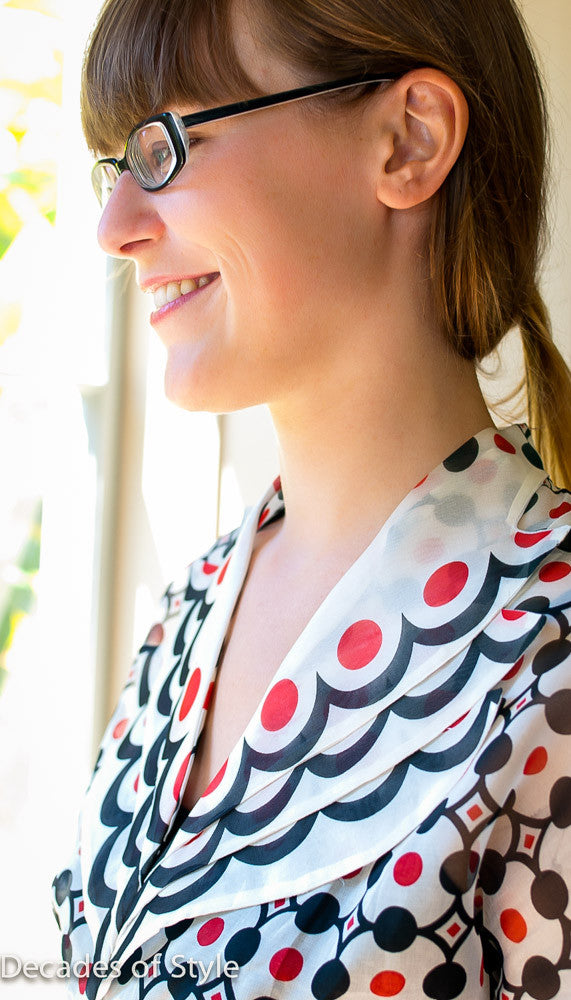The photograph showcases a young brunette woman with her hair pulled back into a ponytail, looking off to the left and smiling. She wears stylish, black, thick-rimmed eyeglasses, suggesting the image is an advertisement for the glasses, especially with the caption "decades of style" in white text at the bottom left corner. She is dressed in a white blouse adorned with red circles and navy blue lines, featuring a v-neck and an artsy pattern. The background is slightly blurred but indicates that sunlight is streaming into the room, hinting at daytime, and a few hints of plant life can be observed. The overall scene suggests a fashion-focused context, possibly from a magazine or photo shoot.